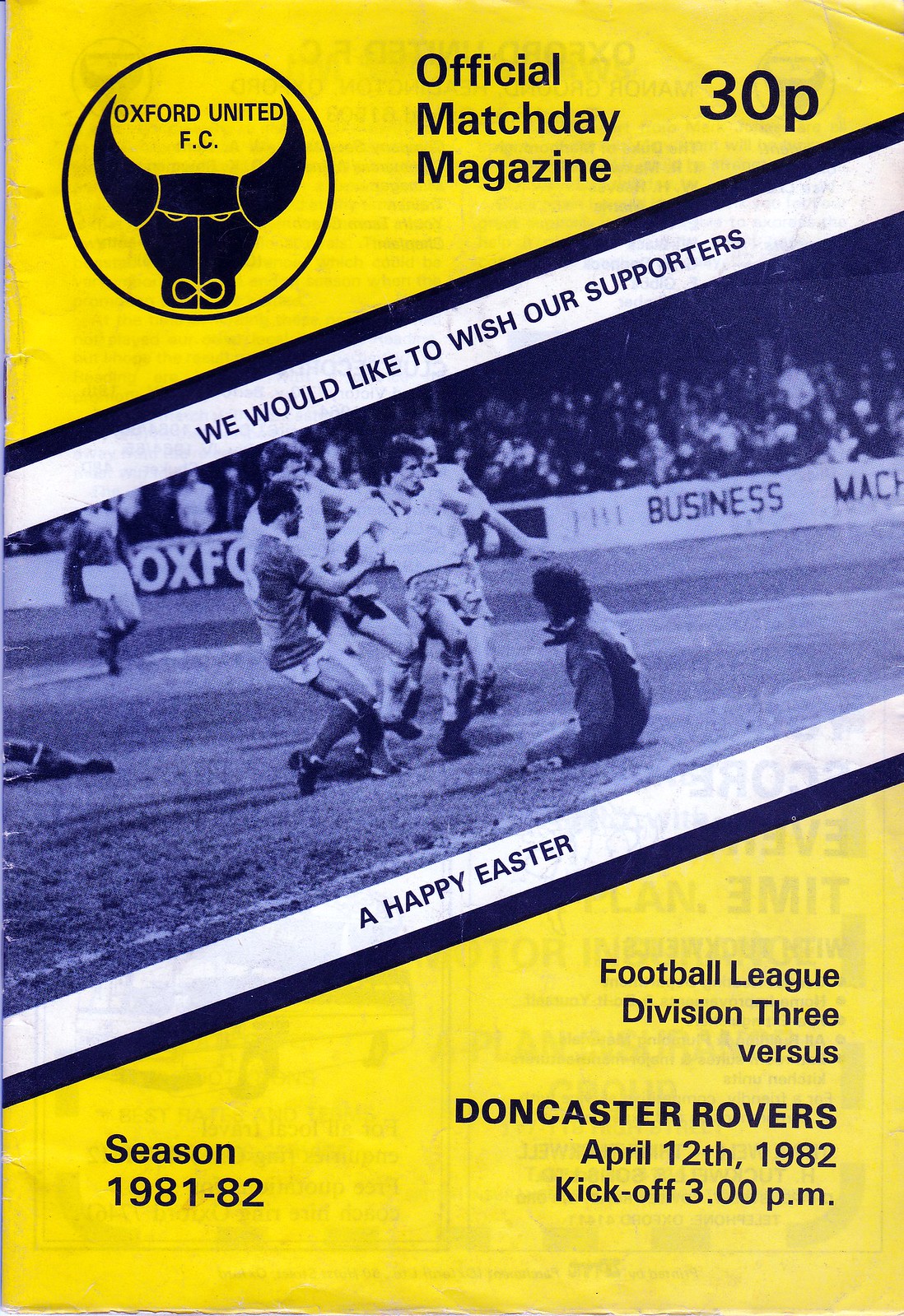The image is a highly detailed cover of a match day program for Oxford United FC. The entire design predominantly features the colors yellow, blue, and white. At the top left of the cover, there's the Oxford United FC logo, depicting a bull's head in black. Directly to the right, it reads "Official Match Day Magazine" with a price tag of 30p. The title is framed by horizontal white bars; the top bar bears the message, "We would like to wish our supporters a Happy Easter," in blue text.

The central part of the cover showcases a tinted blue-toned photograph of football players in the midst of celebrating a goal. Players are seen rushing towards the goal scorer, while the background captures an enthusiastic crowd cheering. There's a mix of strips alternating between blue and white, enhancing the visual structure of the cover.

At the bottom left, the text reads "Season 1981-82" in blue, while on the bottom right, it specifies "Football League Division 3 vs. Doncaster Rovers, April 12th, 1982. Kickoff, 3pm" also in blue.